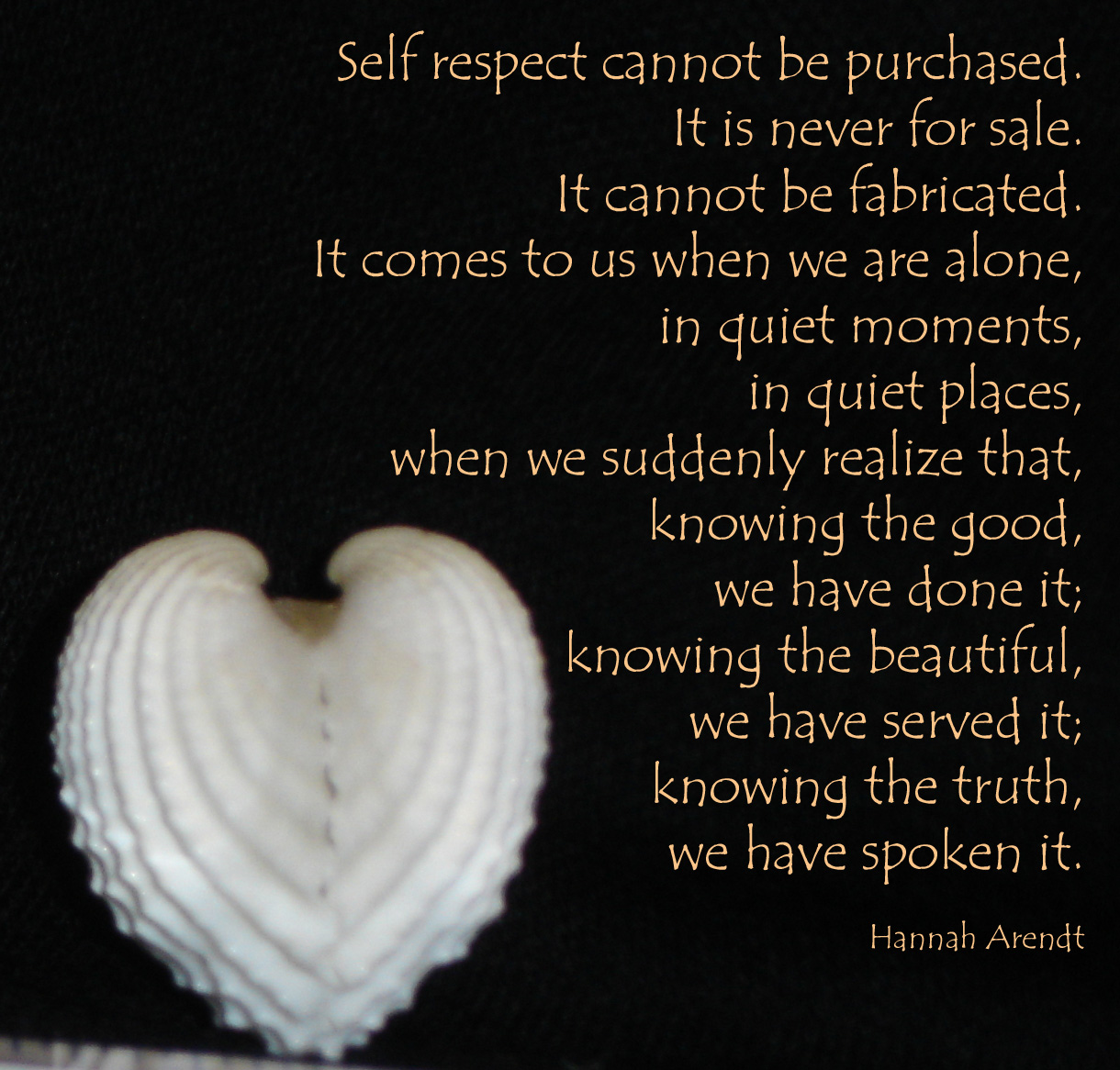On a black square graphic designed for social media, the quote written in orange-yellow text states: "Self-respect cannot be purchased. It is never for sale. It cannot be fabricated. It comes to us when we are alone, in quiet moments, in quiet places, when we suddenly realize that, knowing the good, we have done it; knowing the beautiful, we have served it; knowing the truth, we have spoken it." The quote is attributed to Hannah Arendt. Positioned at the bottom left corner is a slightly blurry, heart-shaped seashell, predominantly white with gray ripples and layers, enhancing the graphic’s contemplative mood. The text is neatly aligned on the right side, adding to the overall aesthetic and clarity of the message.